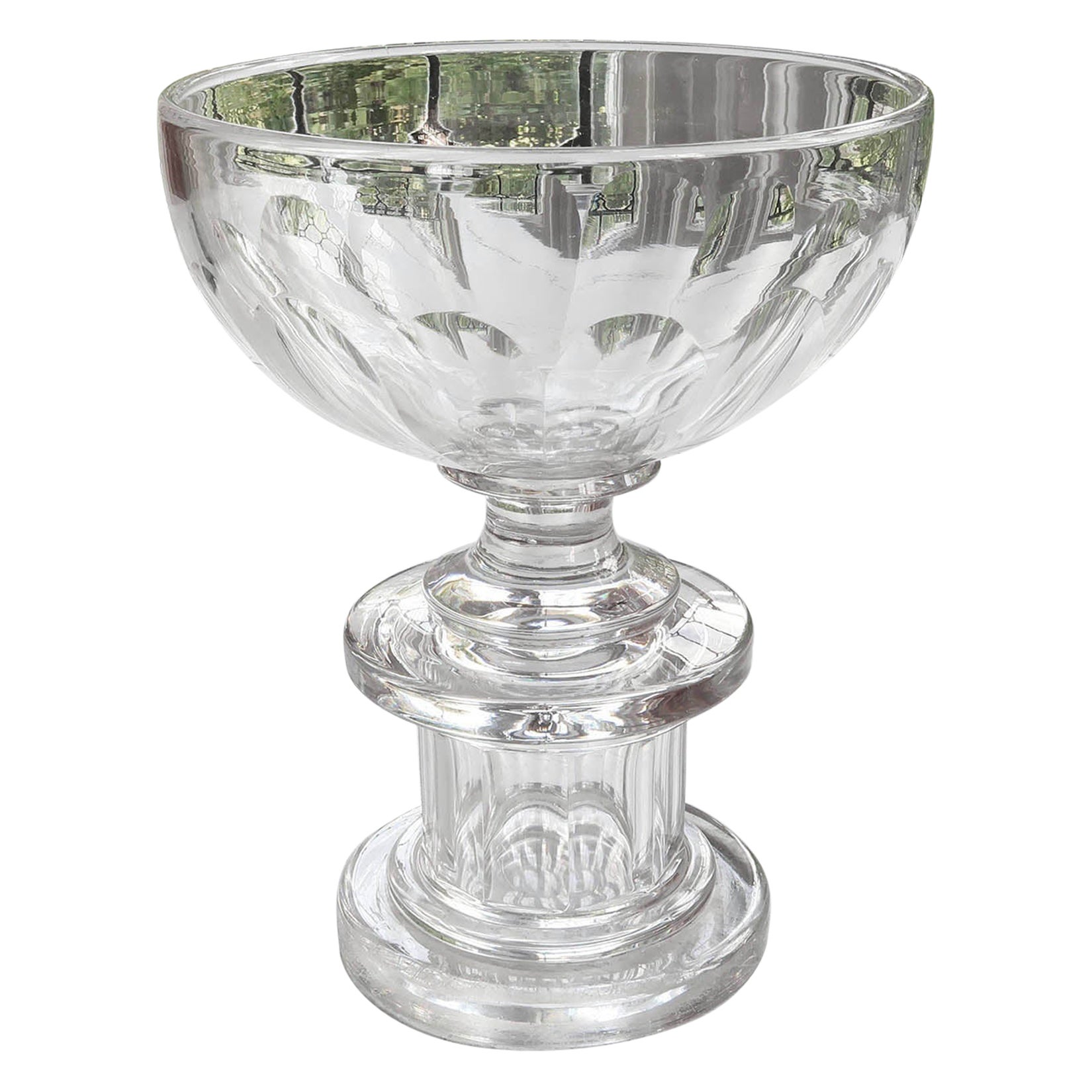The image depicts a crystal-clear, silver-colored chalice, prominently displayed against a plain white background. The chalice features a beautifully ornate stem with intricate etchings, and it is topped by a reflective bowl, approximately three inches in diameter, which captures the serene image of a green garden behind it. The design incorporates multiple circular elements: a smaller base supporting the bowl, followed by a slightly larger base, and an even wider circular base at the bottom. These bases contribute to the chalice's elegant yet not overly extravagant appearance. The piece exudes a refined simplicity that could suggest its use as an ornamental candy dish or a display goblet. Various reflections in the chalice highlight its reflective surface and crystal craftsmanship, emphasizing its delicate, fluted design.